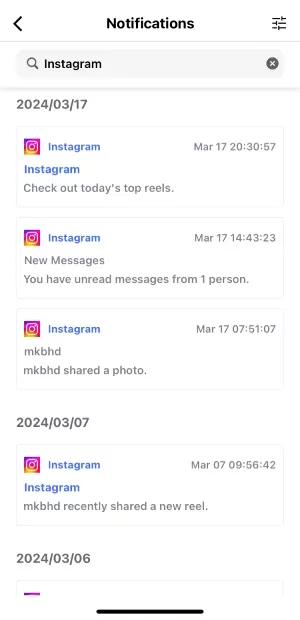This screenshot from a mobile device captures the "Notifications" page, as indicated by the header at the top of the screen. The user interface elements include a back arrow on the upper left, allowing navigation to the previous page, and a settings icon composed of three horizontal lines with configuration knobs on each line on the upper right. Directly below the header is a search bar, displaying the term "Instagram," indicating the notifications listed below are filtered specifically for Instagram.

The notifications are organized by date, following the format year-month-day. The visible dates and their corresponding notifications are as follows:

1. **March 17, 2024:**
   - **Instagram:** Check out today's top reels.
   - **Instagram:** New messages. You have unread messages from one person.
   - **Instagram:** MKBHD shared a photo.

2. **March 7, 2024:**
   - **Instagram:** MKBHD recently shared a new reel.

3. **March 6, 2024:**
   - The notifications for this date are not visible due to the screenshot being cut off at this point, and more notifications would be accessible by scrolling further down the page.

The screenshot does not display the top UI elements of the mobile device, but it offers a clear view of the search-filtered notifications, efficiently organized by date for easy navigation.